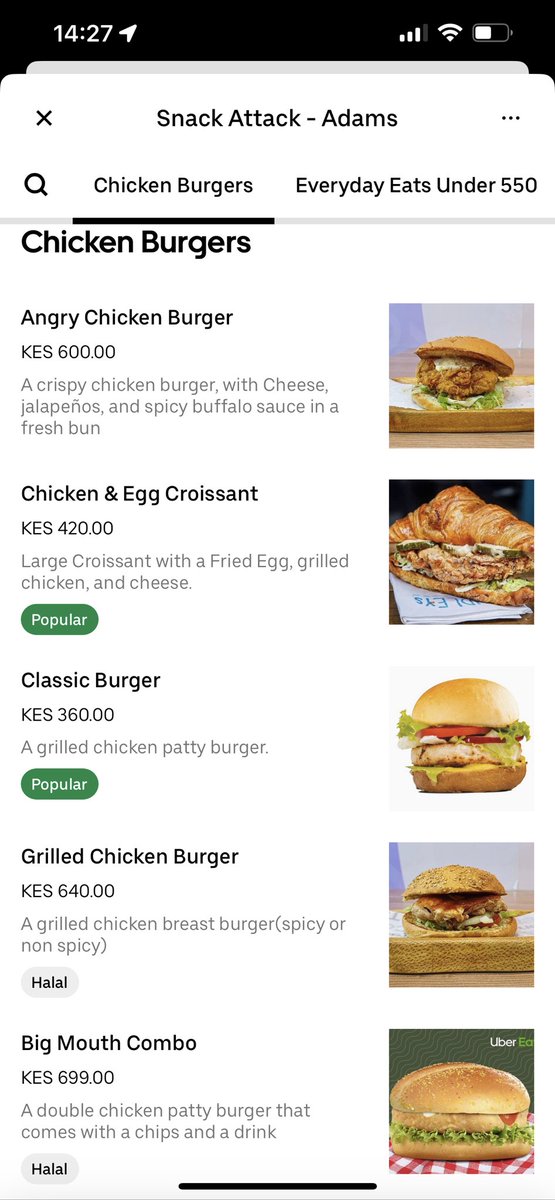The screenshot shows the interface of a food delivery app or a digital menu from a restaurant named "Snack Attack Adams." The time displayed on the phone is 14:27, and the location services symbol is present, indicating the user's location is being tracked. Their phone is connected to Wi-Fi, shows three out of four signal bars, and the battery is approximately 50% charged. 

A pop-up with a close button (an 'X' in the top left corner) and three horizontal dots for more options is visible. The active tab on the menu is titled "Chicken Burgers," and a search function is available on the page. Detailed descriptions of each menu item under this tab include:

1. **Angry Chicken Burger**: Priced at 600 KES (Kenyan Shillings), this item features a crispy chicken burger with cheese, jalapeño, spicy buffalo sauce, served on a fresh bun.
   
2. **Chicken and Egg Croissant**: Priced at 420 KES, this popular item consists of a large croissant filled with a fried egg, grilled chicken, and cheese.

3. **Classic Burger**: Priced at 360 KES, noted as popular, it includes a grilled chicken patty.

4. **Grilled Chicken Burger**: Priced at 640 KES, described as a grilled chicken breast burger available in spicy or non-spicy variations.

5. **Big Mouth Combo**: Priced at 699 KES, this combo includes a double chicken patty burger with chips and a drink.

There is an additional tab labeled "Everyday Eats Under 550 KES", although no further details about this tab are provided in the screenshot.